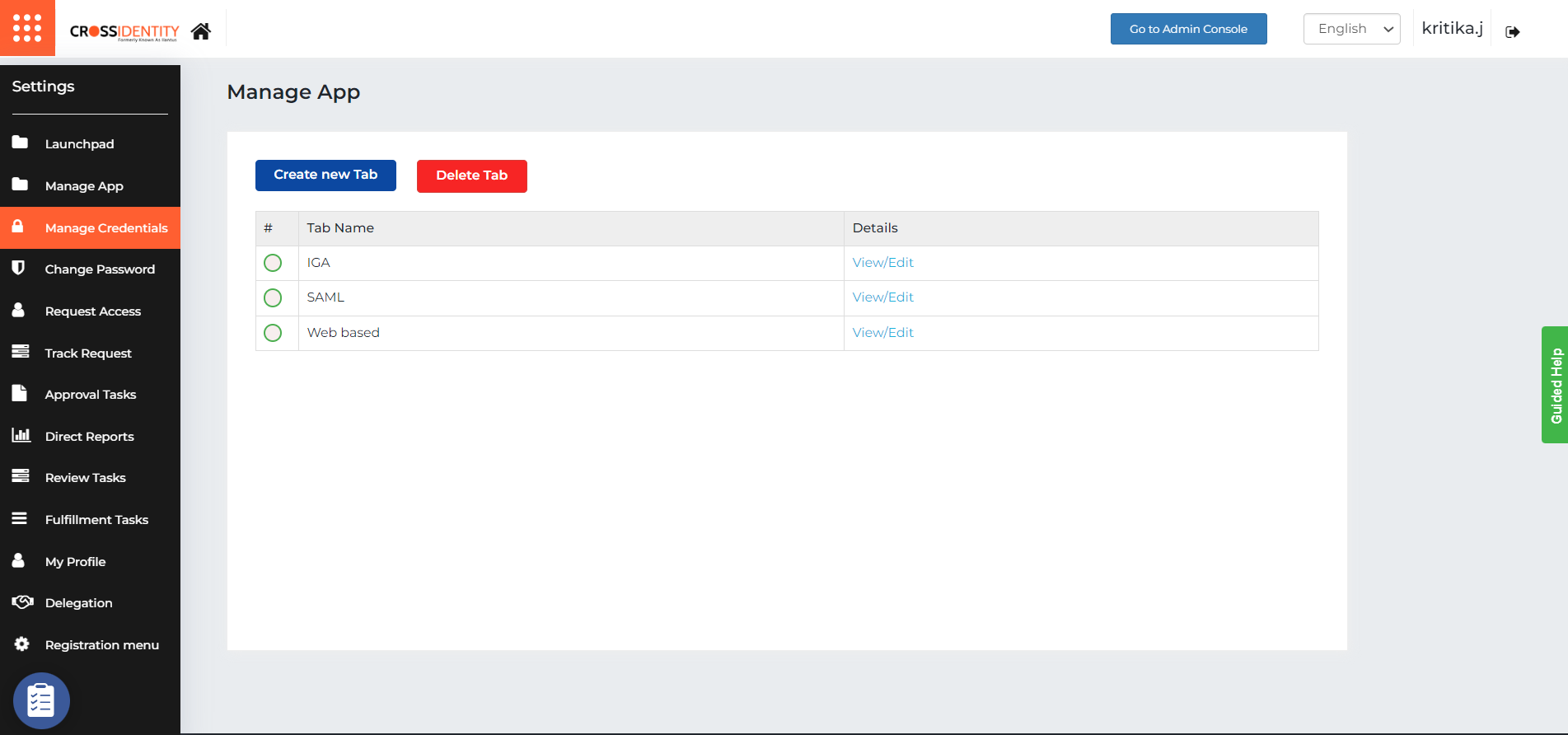This image is a detailed screenshot of a user interface, possibly of a web application or online platform. 

In the top left corner, there's an orange box containing a 3x3 grid of white dots. The label "Cross Identity" is adjacent to it, where "Cross" is in black text and "Identity" in orange. Next to this, there's a home icon.

Along the top banner, which has a white background, there's a blue button labeled "Go to Admin Console," followed by a drop-down language selection menu displaying "English." Further to the right, there's likely the username of the logged-in user alongside a login/logout button.

The main content of the page is structured beneath this top banner. On the left, there's a sidebar with a dark background and white text, listing various options: Settings, Launchpad, Manage App, Manage Credentials, Change Password, Request Access, Check Request, Approval Test, Direct Reports, Review Tasks, Fulfillment Tasks, My Profile, Delegation, and Registration Menu. At the bottom of this sidebar, there is a blue circular icon featuring a clipboard.

The "Manage Credentials" option is selected, highlighted with an orange background instead of the dark background used for the other options.

In the content area titled "Manage App," which has a light gray background, there is a central white box. This box contains a blue button labeled "Create New Tab" and a red button labeled "Delete Tab." Below these buttons is a table with three columns: a numbered column featuring empty circles, a "Tab Name" column, and a "Details" column. 

The table includes three rows:
1. "IGA View/Edit"
2. "SAML View/Edit"
3. "Web-Based View/Edit"

On the right side of the page, there's a green box with white text that reads "Guided Help."